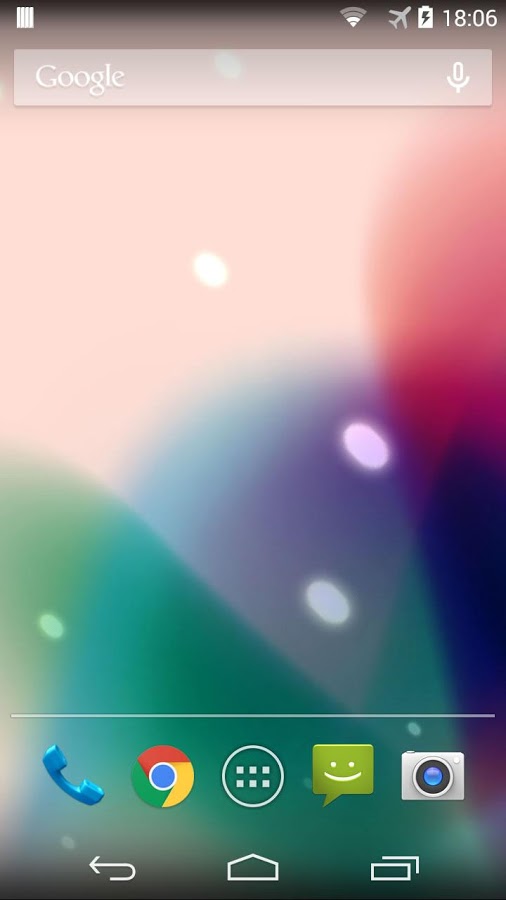Screenshot of an Android phone home screen

The screenshot depicts the home screen of an Android phone, evidenced by the unfamiliar suite of icons and tools to an iPhone user. The screen features a colorful background with green, blue, and red spotlights that fade into each other. White spots resembling headlights are scattered across the background. The status bar at the top shows low Wi-Fi connectivity with two out of five bars and a charging battery indicator. The time displayed is 6:06. 

Dominating the top of the screen is a Google search bar accompanied by a microphone icon to enable voice searches. 

At the bottom, a row of commonly-used app icons is visible:
- A blue phone icon, likely for dialing.
- A circular Google Chrome icon, characterized by its red, yellow, and green outer circle and blue center.
- An icon consisting of six dots within a circle, potentially for app navigation or menu access.
- A green messaging icon with a smiley face.
- A gray camera icon featuring a blue light.
  
Below these app icons, there are three navigation buttons:
- A back button.
- A home button.
- A recent apps button depicted by two stacked boxes.